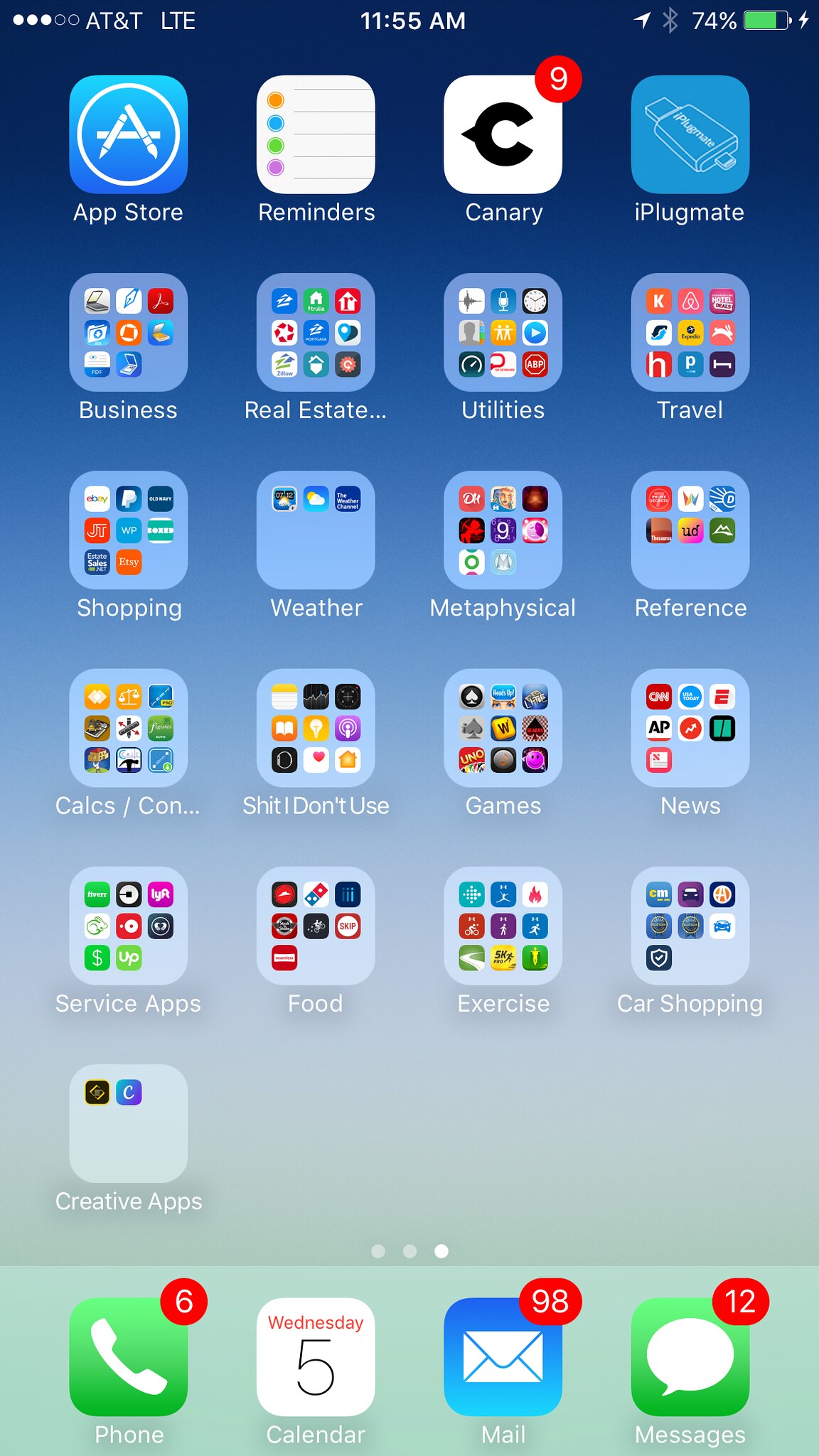This photograph showcases a smartphone screen with a gradient background transitioning from blue at the top to a very light blue-gray at the bottom. The screen is organized into five rows of four icons each, with an additional single icon at the bottom of the main portion of the screen. Below these icons are three dots, with the far-right dot highlighted in white while the others are gray, indicating the current page of the home screen.

At the very bottom, set within a slightly blue-green border, are four more icons. On the far left is a green telephone icon labeled "Phone," which features a red notification badge with the number 6. Next is a white calendar icon with the text "Wednesday" in red and the number 5 in black, labeled "Calendar" beneath the icon. The third icon is a blue envelope symbolizing "Mail," accompanied by a red notification badge displaying the number 98. Finally, to the right is a green speech bubble icon labeled "Messages," with a red notification badge showing the number 12.

Each icon is square with slightly rounded corners, maintaining a consistent and organized appearance across the screen.